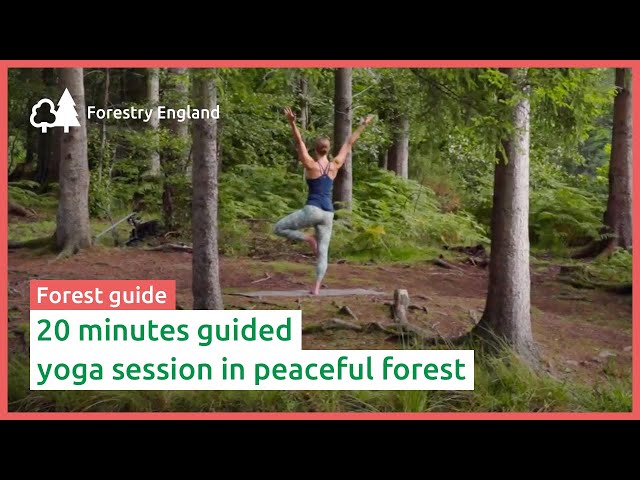The image captures a serene forest scene framed by a pink rectangular border with black bars at the top and bottom. Text overlays include "Forestry England" with an accompanying logo of two stylized trees in the top left corner, and "Forest Guide" along with "20 Minutes Guided Yoga Session in Peaceful Forest" in white and green text at the bottom.

In the center of the image stands a woman on a yoga mat within a clearing surrounded by tall, green trees and bushes. She is performing a yoga pose, balancing on her right leg while her left leg is bent with her foot resting against her inner thigh, forming a tree pose. Her arms are extended upwards in a V shape. She is dressed in a blue tank top with spaghetti straps and light gray yoga pants. The ground is flat and interspersed with patches of grass and dirt, and some fallen branches are visible in the background. The photograph, taken during daylight, showcases a peaceful, natural setting ideal for the guided yoga session being advertised.